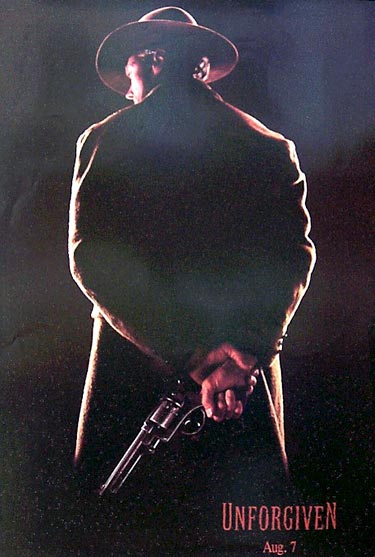The image is a striking poster, presumably for an event or a movie titled "UNFORGIVEN," taking place on August 7th. The poster prominently features a lone man, depicted from behind, dressed in a long, possibly brown duster coat typical of the Old West and a wide-brimmed cowboy hat of a similar shade. His posture is rigid and imposing, with his left hand gripping his right wrist behind his back, where he also discreetly holds a sizable revolver, reminiscent of a Colt .45. The backdrop is a somber black, accentuating the serious and dramatic tone of the image. The lower right corner of the poster prominently displays the title "UNFORGIVEN" in bold, pinkish-red capital letters, with the date "AUG. 7" directly below it in a similar font. The overall color scheme of the poster includes various shades of brown and pink, adding to the vintage western aesthetic.